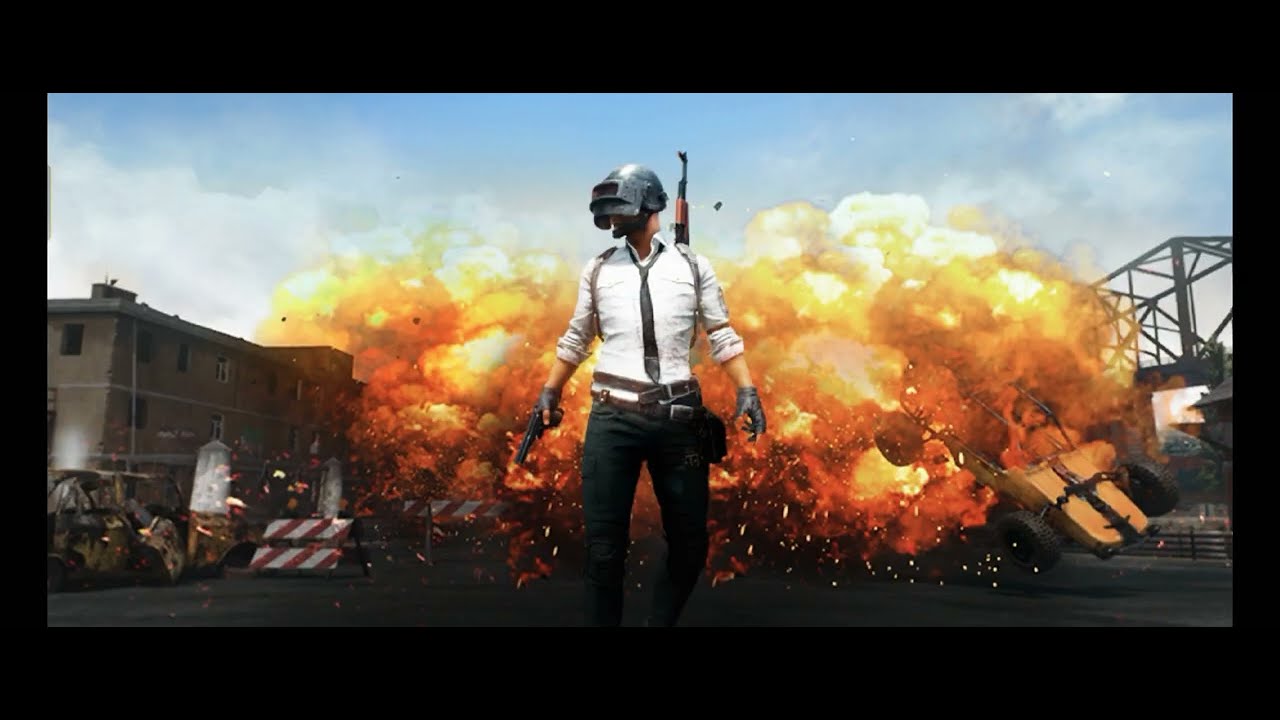The image, framed with a thin black border, depicts a hyper-realistic, stylized scene resembling a video game or graphic art. At the center stands a well-dressed man, clad in a long-sleeve white button-up shirt, black tie, and black pants. His ensemble is completed with black gloves, a belt, and a helmet that covers his head and face, evoking a futuristic or virtual reality headset. He carries a handgun in his right hand and a rifle strapped across his back. He stands against a dramatic backdrop of a large explosion, with billowing reddish-orange smoke, and a partially visible dune buggy being blown apart by the blast. On the left side of the frame, there are cautionary stop signs and signs of buildings, while the right side shows what appears to be a metal bridge with some blue sky visible above. The tableau is reminiscent of a cinematic action sequence.